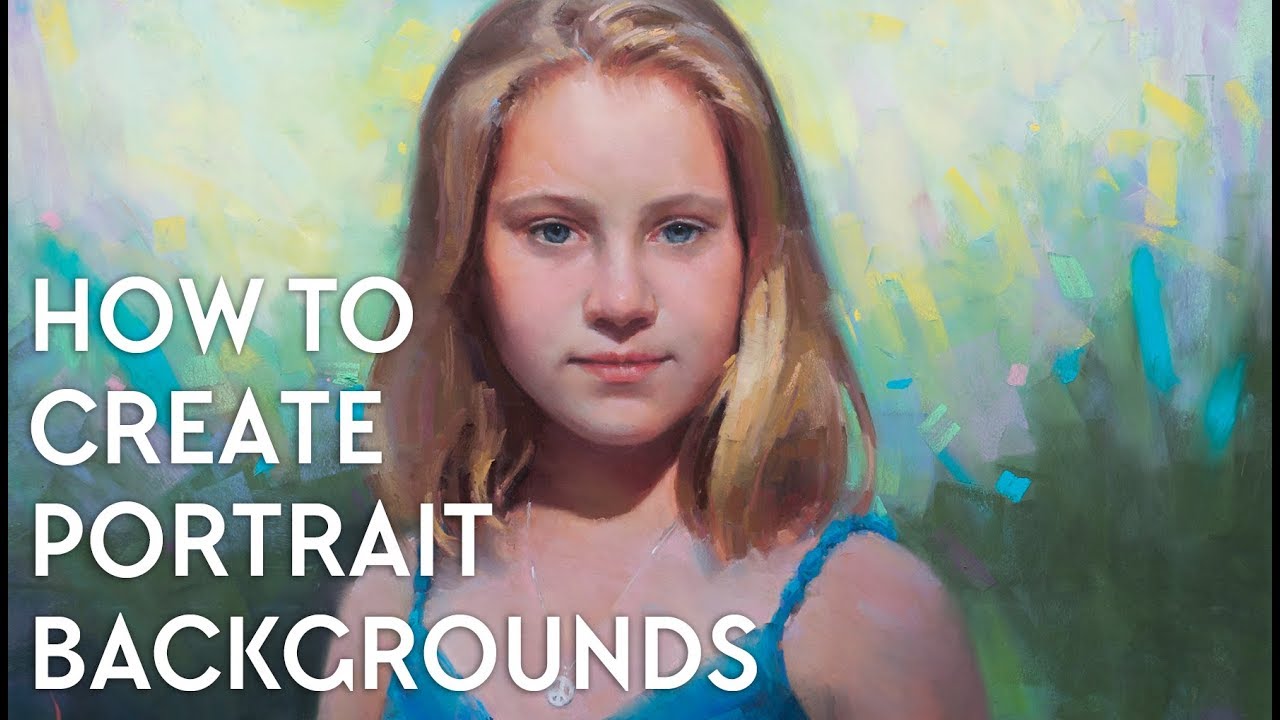The image is a horizontally rectangular, multi-color painting with digital elements, framed by a thin black border on the left, right, and bottom edges. The background features a rich array of pastel colors with light blue, yellow, lavender, and touches of pink brush strokes scattered in various directions. The lower third of this painting is dominated by dark green vertical brush strokes.

At the center, a young blonde-haired girl with shoulder-length hair and blue eyes is portrayed looking directly at the viewer, her face without expression. She is wearing a blue spaghetti strap top and a silver necklace.

White, all-capital letters in a centered, descending stack along the left side of the image read: "HOW TO CREATE PORTRAIT BACKGROUNDS." This stylized text emphasizes the instructional theme of the artwork, suggesting that the depicted background can be created by following the provided guide.